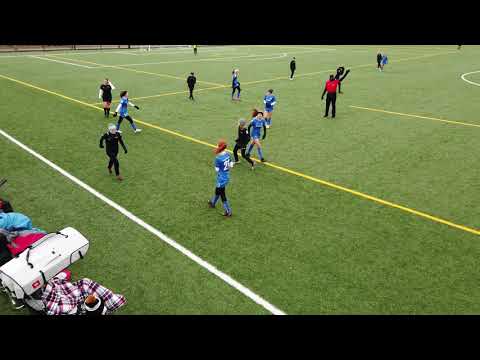This detailed image captures a moment during what appears to be a soccer game, although the action is paused with players milling around. It's a tight shot focusing on a section of the grassy field, marked with white and yellow lines. In the foreground, the bottom left corner is cluttered with personal belongings, including clothing and bags, seemingly piled on a bench. The players, primarily in blue uniforms, are scattered across the field and sidelines, some standing and others walking, suggesting either a break or practice session. Among them, players in black uniforms can also be seen, likely the opposing team. A man in a red shirt and black pants, possibly a referee, stands out in the midst of the field. The mood is relaxed, as no game action is currently underway, and the soccer ball is not visible, potentially obscured near a player's foot.